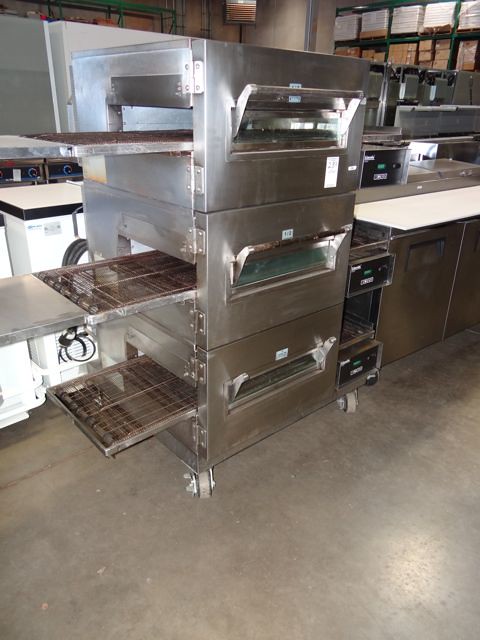A colored photograph captures the scene of what appears to be an industrial kitchen or kitchen warehouse, characterized by tall, industrial shelves like those at Home Depot, laden with boxes and possibly other equipment stacked up. Dominating the foreground are three rusted metal conveyor-belt ovens, likely used for baking pastries or pizzas, stacked vertically. Each oven is equipped with a metal conveyor belt designed to pull uncooked items through the heating process until they emerge cooked. The conveyor belts are notably rusted, adding a worn appearance to the setup. Each oven features a small viewing window to monitor the baking process, and a large handle on the right side for operation. To the right of these ovens, partially visible, is what appears to be a blurry control panel with a green light or button. The entire contraption rests on a concrete gray industrial flooring, enhancing the utilitarian feel. Behind the ovens, there are additional white appliances that are somewhat indistinct, possibly including a washing machine. The background reveals green shelves filled with plastic-wrapped boxes and other warehouse items. The angle of the photograph contributes to the complexity of the scene, providing a glimpse into a busy, multifaceted industrial workspace.